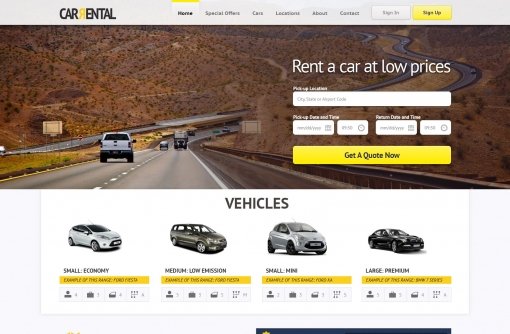The image features a light purple background at the top, prominently displaying the text "Car Rental" with a yellow "R" beside it. Above the yellow "R," there is a small yellow line marked "Home." There are additional headings, including "Special Effects" and "Cars," alongside a few smaller, less legible labels. On the right side, buttons for "Sign In" and "Sign Up" are visibly colored in yellow.

Beneath this section, the background transitions to a darker shade, featuring a scenic highway cutting through mountain terrain, bustling with numerous cars. To the right of this highway image, bold text reads "Rent a Car at Low Prices," followed by a search block with options to input times and dates for vehicle pickup. A prominent yellow button labeled "Get a Quote Now" is positioned below this search block.

Under the highway imagery, a dropdown white box showcases various vehicle options:
1. "Small Economy" with a yellow button beneath it and accompanied by four small icons.
2. "Medium Low Emission," also featuring a yellow button and similar icons.
3. "Small NM" with a yellow button and four icons.
4. "Large Medium," again with a yellow button and accompanying icons.

Alongside these options, a blue box is visible with a tiny red spot located at its lower left corner. Adjacent to this blue box is a long black line with a small, rounded spot on its left end.